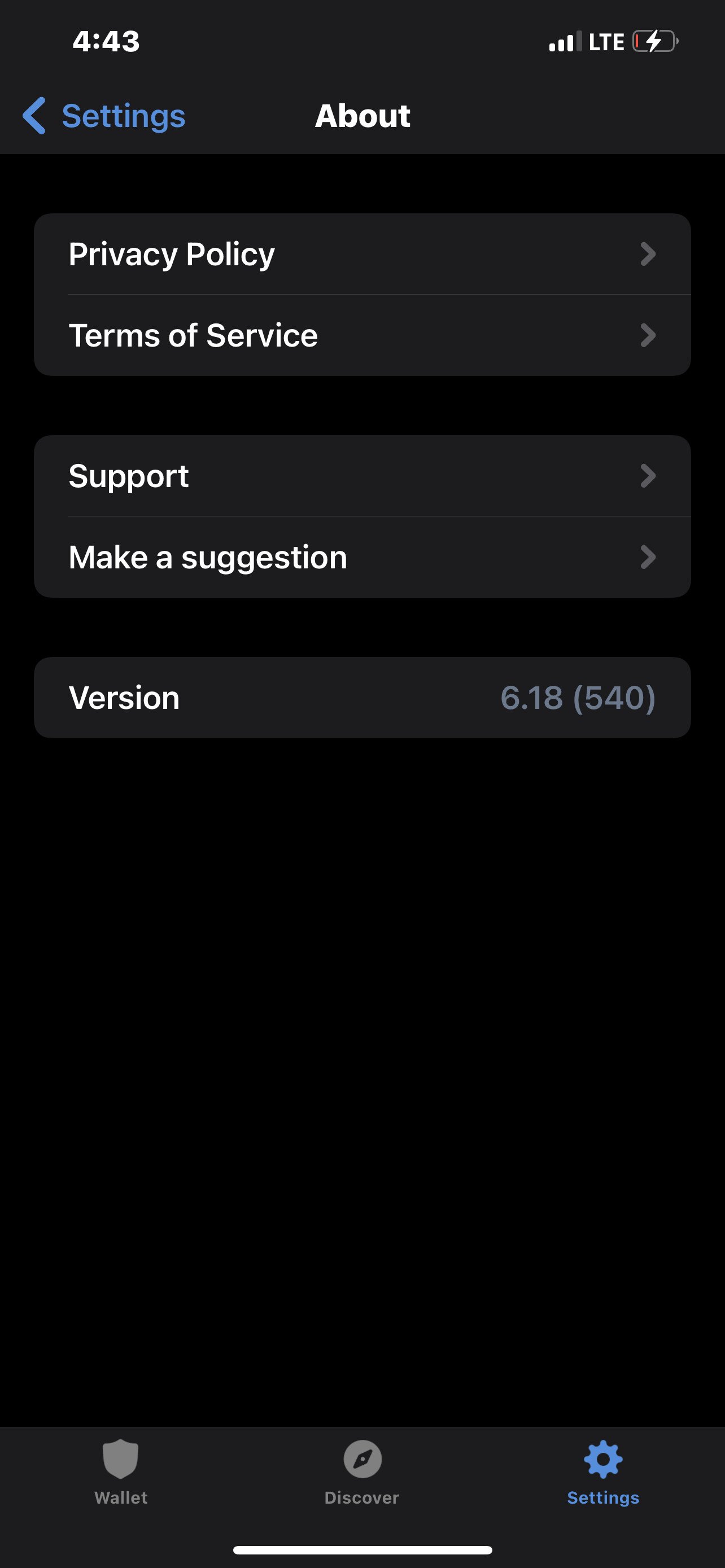**Detailed Settings Page Screenshot Description:**

The screenshot captures the settings page of a smartphone interface. At the very top, the status bar shows the time as "4:43," along with three to four signal bars and an "LTE" indicator, suggesting a strong cellular connection. Adjacent to the signal indicator, there is a battery icon lying on its side. The battery meter features a nearly invisible red bar, indicating that the battery is almost dead. However, the presence of a lightning bolt symbol across the battery icon suggests that the device is currently being charged.

Below the status bar, the screen displays a header titled "Settings" with a blue, left-pointing back arrow beside it. The main section of the screen, set against a dark gray background, contains three lighter gray rectangles.

1. **First Rectangle:**
   - Displays two lines of text:
     - "Privacy Policy"
     - "Terms of Service"
   - Both texts are in white, each accompanied by a gray arrow pointing to the right, separated by a thin gray line.

2. **Second Rectangle:**
   - Features two options:
     - "Support"
     - "Make a Suggestion"
   - Similar design to the first rectangle with white text, gray right-pointing arrows, and a gray dividing line.

3. **Third Rectangle:**
   - Contains a single line of text:
     - "Version" in white text
   - To the right, it displays "6.18" in light blue font, followed by "[540]" in brackets, with no arrow present.

At the very bottom of the screen, there's a navigation bar with four icons:
   - A shield labeled "Wallet"
   - A compass labeled "Discover"
   - A blue gear labeled "Settings" (highlighted to indicate the current section)

This detailed description encapsulates the entire interface and functionality seen within the screenshot.